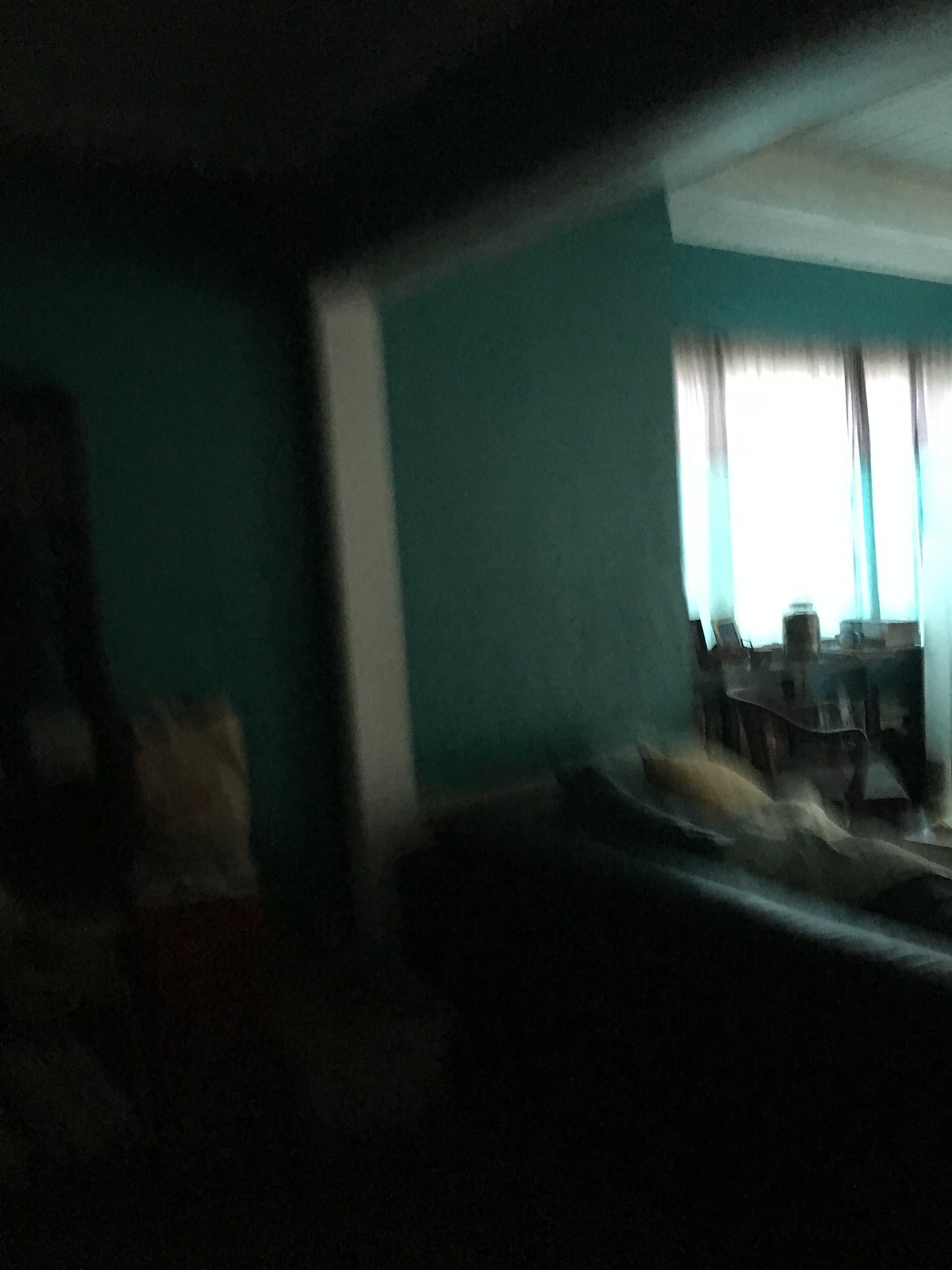The photo is an out-of-focus image taken in a dark room within a home, characterized by its indistinct details. Even with the blur, elements of the room's layout and some specifics can be discerned. The walls are painted a turquoise or aqua color, and there is a white door frame that opens into a larger room, possibly a living room. Light filters into this adjacent room through big windows adorned with sheer curtains. In the foreground, there is a long couch with cushions, though the material is unclear. On the right-hand side of the photo, a chair appears to be positioned near a piece of furniture resembling a bookshelf or shelving unit, which holds various knickknacks. The room is dark overall, with some areas better lit by natural light coming from the windows in the larger adjoining room.